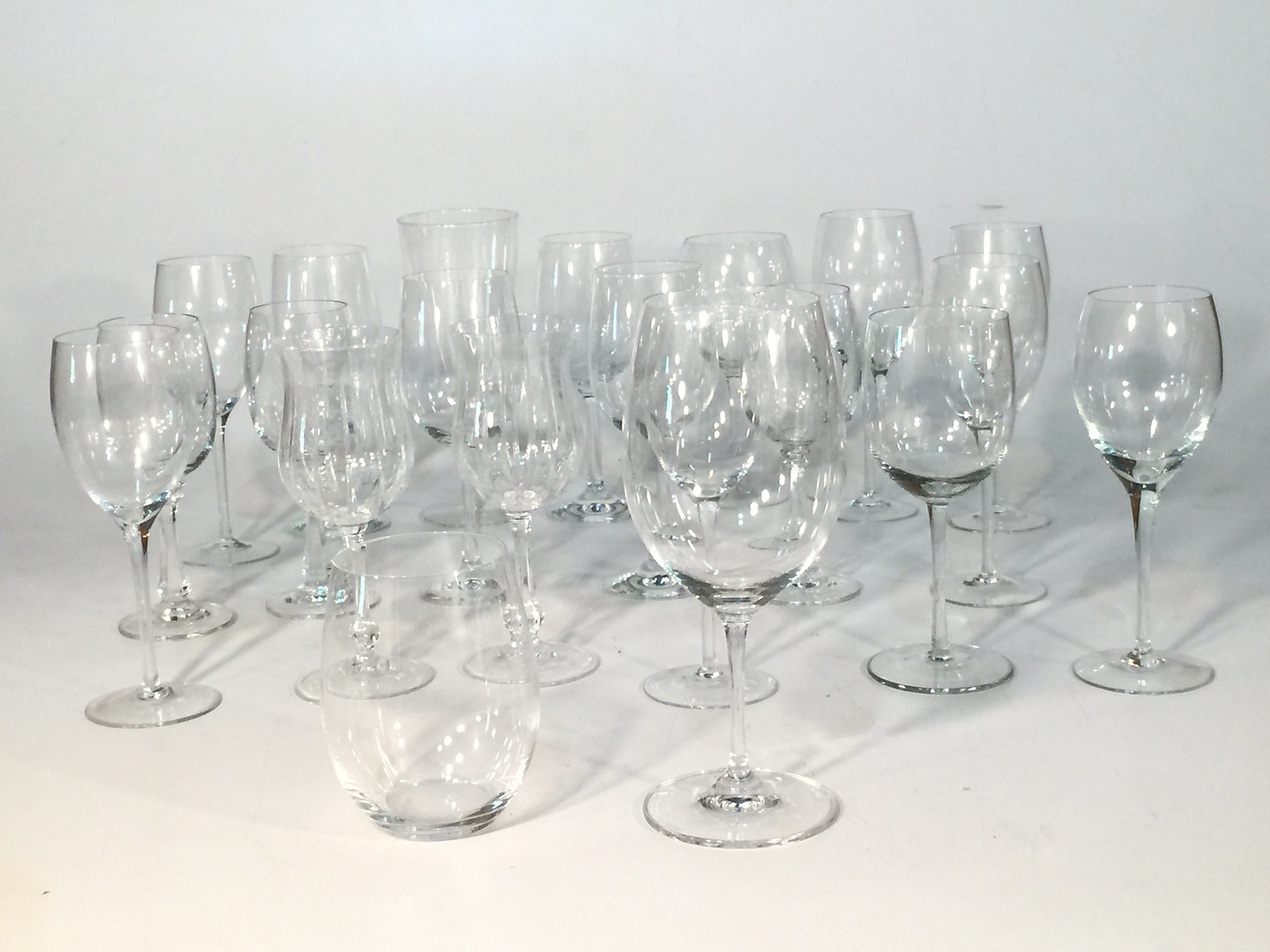This monochromatic photograph features an array of various glassware, predominantly wine glasses, arranged on a cream-colored surface against a backdrop that transitions from light gray at the top to tan at the bottom. The densely packed glassware includes a diverse assortment of shapes and sizes: tall and wide wine glasses, narrower and semi-tall ones, several stemmed wine glasses, and a stemless tumbler positioned near the front. One glass at the back, appearing to have a wide mouth and a straight down edge, is partially obscured by another glass in front of it. The glasses are clear, reflecting the background and casting intricate, overlapping shadows on the surface. The lighting, emanating from both sides, accentuates the clarity and shininess of the glassware, creating an interplay of light and shadows that lends depth to the composition.